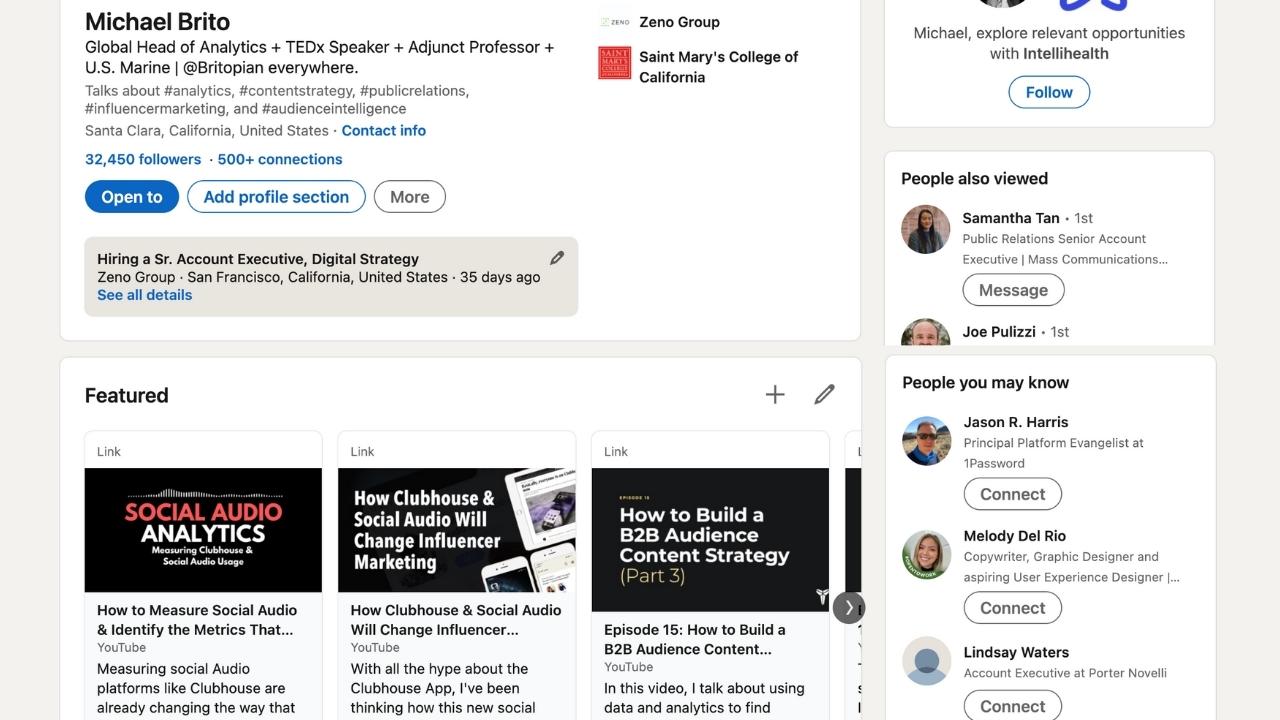A screenshot of a professional networking website, likely LinkedIn, displays the profile of Michael Brito. His title reads "Global Head of Analytics, TEDx Speaker, Adjunct Professor, and US Marine." His self-description covers expertise in analytics, content strategy, public relations, influencer marketing, and audience intelligence, using hashtags for emphasis. Michael is based in Santa Clara, California, United States, and boasts 32,450 followers along with over 500 connections.

The profile notes that Michael is actively hiring for a Senior Account Executive in Digital Strategy at Xeno Group, located in San Francisco, California—a position listed 35 days ago. 

Suggested connections include Jason R. Harris, Principal Platform Evangelist; Melody Dale Rio, Copywriter, Graphic Designer, and Aspiring User Experience Designer; and Lindsay Waters, Account Executive at Porter Novelli. Viewers also viewed Samantha Tan, a Senior Accountant in Public Relations, and Joe Pulizzi.

Three prominent advertisements with links are featured in the bottom left corner of the webpage.